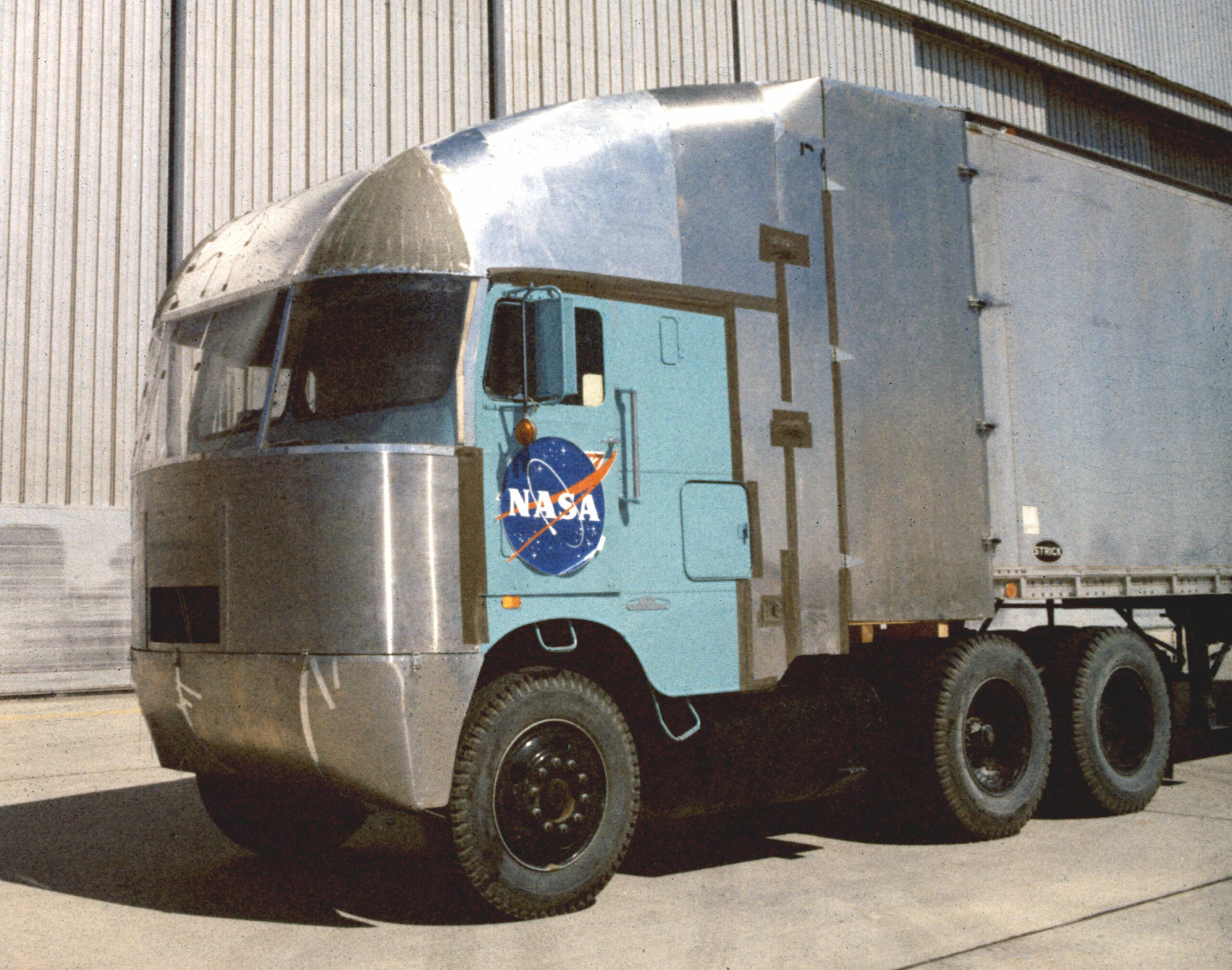This detailed image features a NASA tractor trailer, showcasing a distinctive blend of colors and designs. The cab of the truck is painted in an aqua blue with a prominent NASA logo adorned on the side. This logo includes a large world symbol encircled with orange rotational marks and the letters "NASA" prominently displayed. The front end of the truck is silver, polished to a reflective sheen, contrasting with the more muted silver of the trailer compartment, which is less reflective.

The aerodynamic cab is an unusual design for a truck, with an elongated and streamlined front, distinguishing it from the typically boxy fronts of traditional tractor trailers. The windshield of the truck extends forward, enhancing its aerodynamic profile.

The photo was taken on a sunny day, as indicated by the shadows on the ground and the reflections on the truck's polished surfaces. The truck is parked in front of a large silver hangar, not inside a warehouse or garage as it initially may seem. There is no one visible inside the truck or around it in the photo. The setting and the design of the truck suggest it may be a vintage model, possibly from several decades ago, which adds to its unique charm.